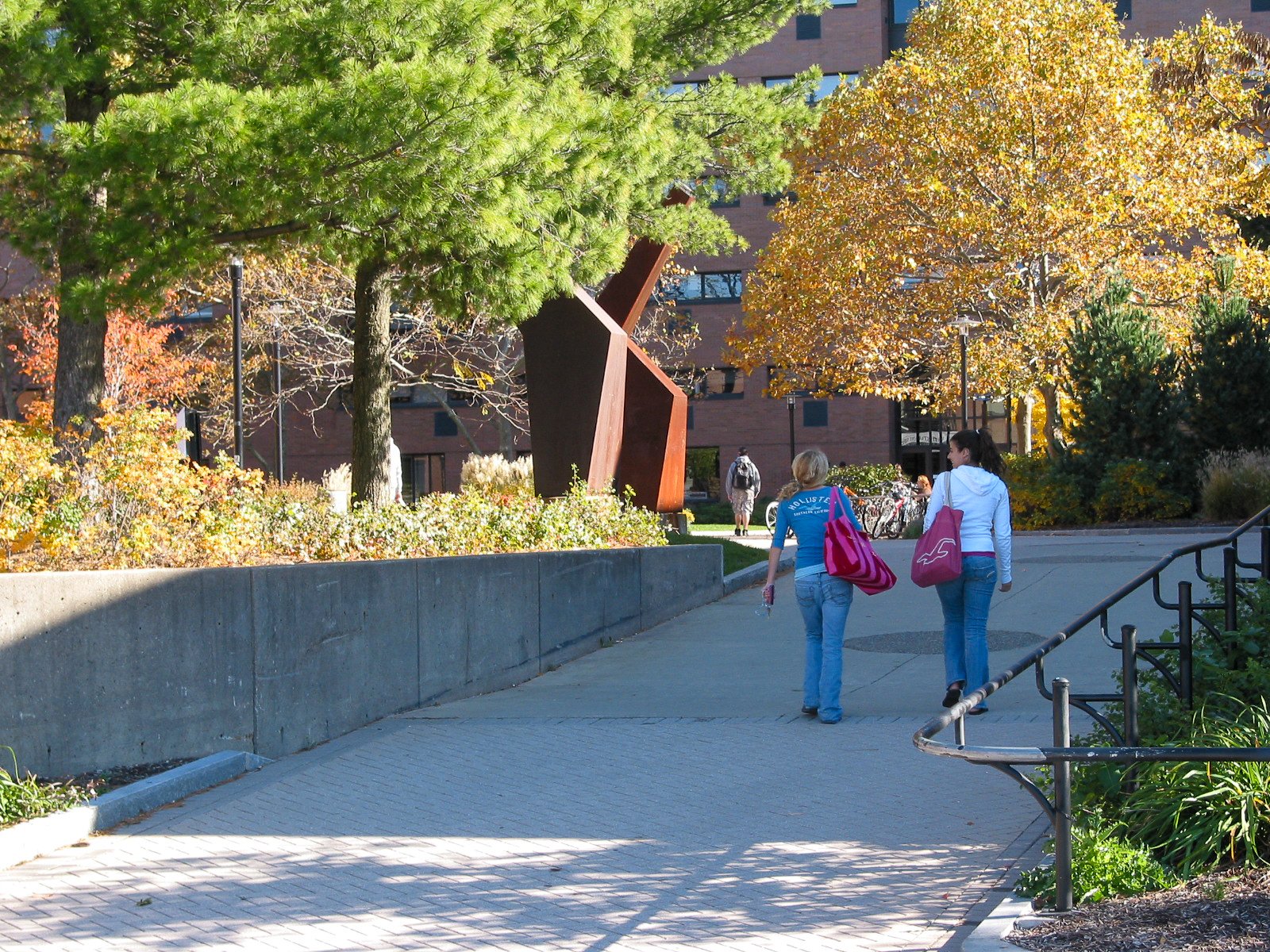This photograph, taken on a bright, sunny day in the fall, captures a scene on a college campus. In the foreground, two college-aged girls are walking on a long concrete walkway flanked by a metal railway that dips into the ground, revealing a small garden area. To the left of the walkway, there is a concrete wall topped with a series of bushes and trees, with their leaves turning orange and yellow.

The girl on the right is wearing blue jeans and a white sweater, her brown hair tied back in a ponytail. She carries a pink bag on her shoulder that features a logo with a bird. To her left, her friend with blonde hair also tied in a ponytail wears a blue, full-sleeve shirt with "Hollister" written on the back and blue jeans as well. She has a larger, red and pink duffel bag slung over her right shoulder. 

Further in the distance, a man with a backpack walks towards a school building that occupies most of the background. The building, identified by a logo, is surrounded by more bushes and trees, adding to the picturesque autumn landscape.